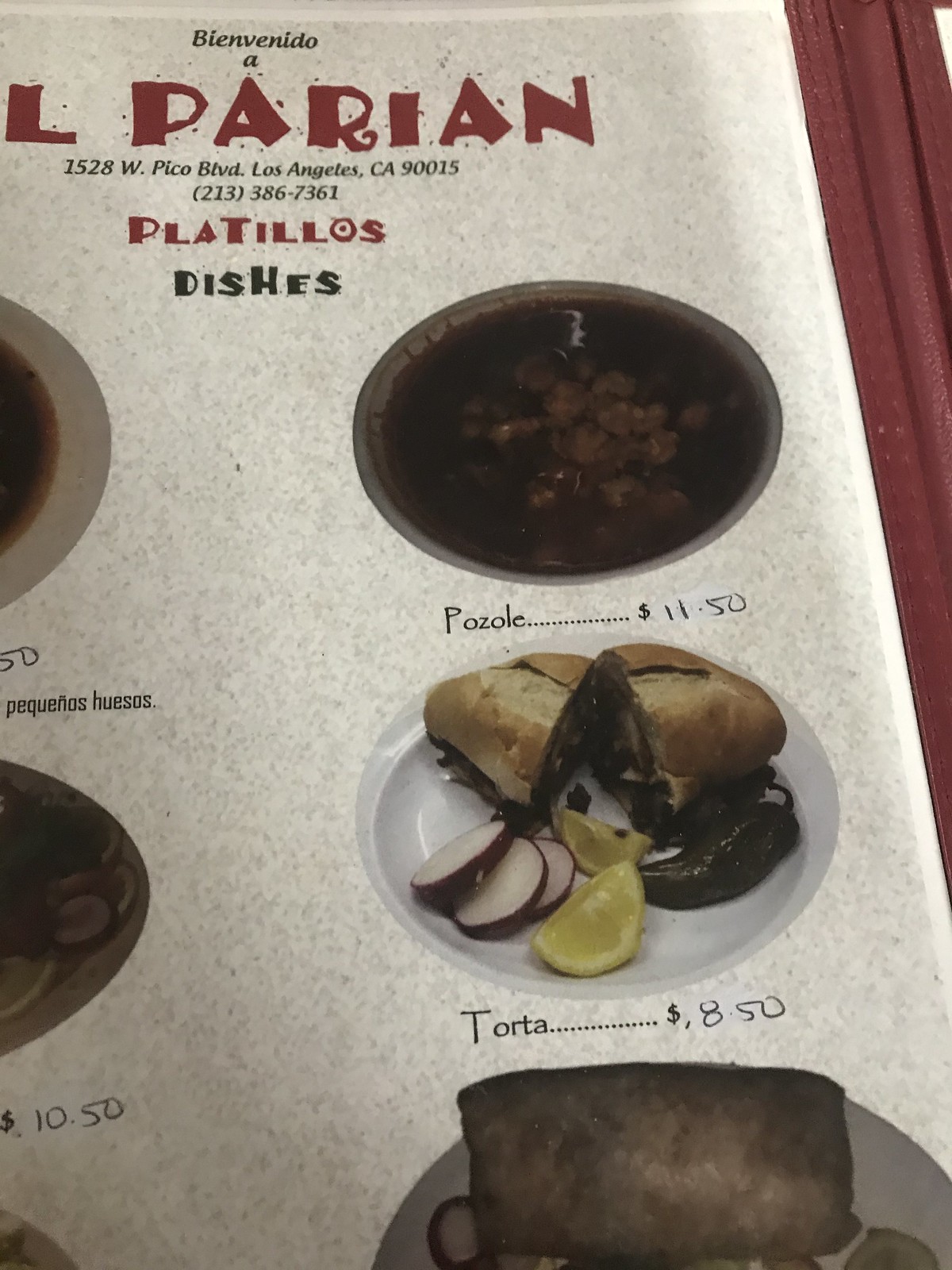Detailed and Descriptive Caption:

"This image showcases a menu from Bienvenido El Perrin, a restaurant located at 1528 West Pico Boulevard, Los Angeles, CA 90015. The menu lists a variety of dishes, including Pozole priced at $11.50 and Torta at $8.50. Unfortunately, some of the other menu items are not clearly visible in the photograph. For further inquiries or to place an order, the restaurant's contact number is 213-386-7361."